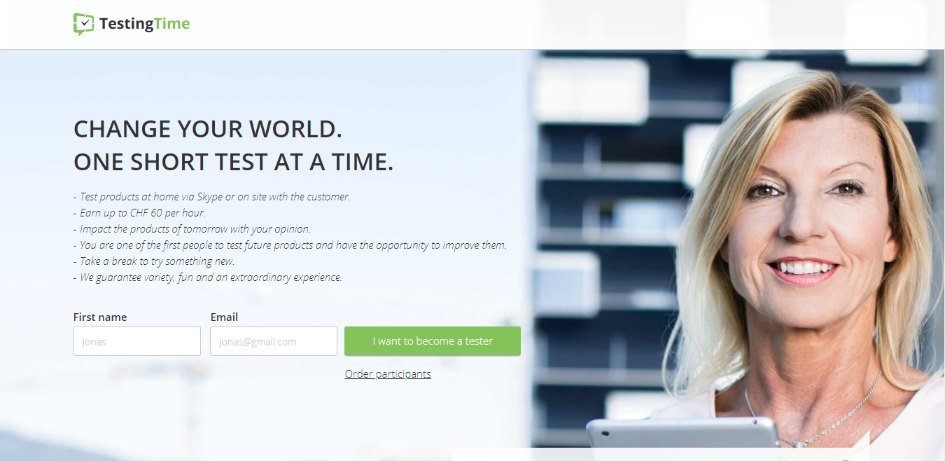This image displays a webpage for a product testing platform named "Testing Time." The page header prominently features the title "Testing Time," with "Testing" written in black and "Time" in green, accompanied by a logo consisting of a green square with a black checkmark centered inside it.

Beneath the header, motivational text reads: "Change your world. One short test at a time. Test products at home via Skype or on-site with a customer. Earn up to CHF 60 per hour. Impact the products of tomorrow with your opinion. You are one of the first people to test future products and have the opportunity to improve them. Take a break to try something new. We guarantee variety, fun, and an extraordinary experience."

A form is shown with a placeholder for a first name, currently displaying "Jonas," and an email field with the placeholder "jonas@gmail.com." Below the form is a green button that reads "I want to become a tester."

Additionally, there is a photo of a smiling woman with blonde hair holding a tablet, suggesting she might be a user of the platform. The background features white walls and light fixtures, creating a modern and inviting atmosphere. The webpage’s color scheme primarily consists of light blue and white, giving it a clean and professional look.